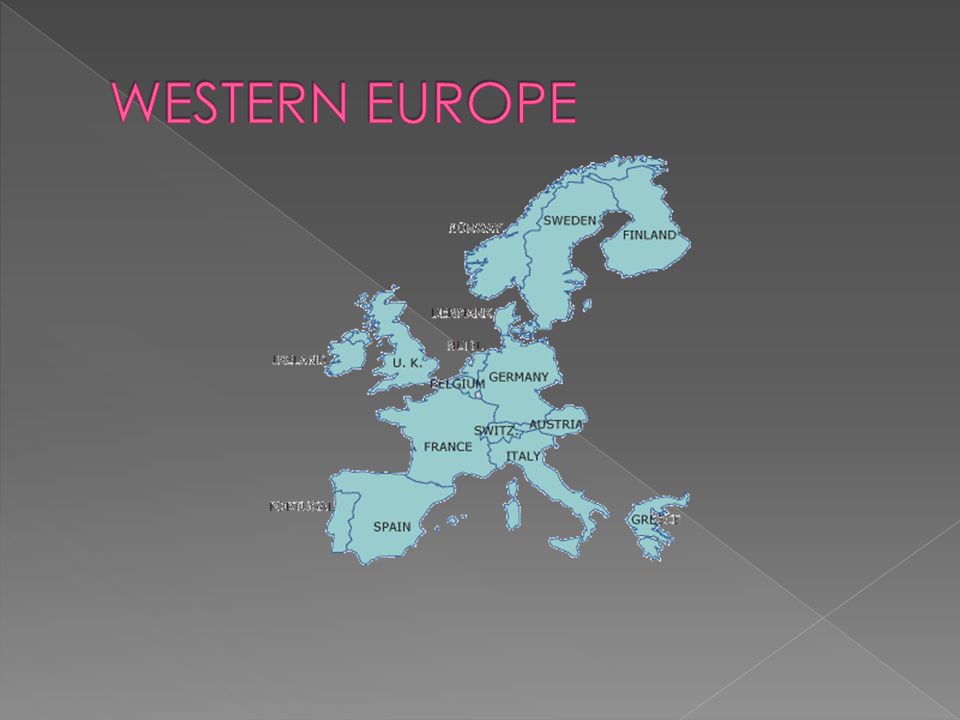The image is a horizontal, rectangular map focused solely on Western Europe against a dark gray background that is diagonally divided, with the upper right corner being a darker shade and the lower left a lighter gray. At the top left of the image, large, hot pink capital letters spell out "WESTERN EUROPE." Beneath this title and occupying the center of the image is a detailed map of Western Europe. The countries, highlighted in a teal or turquoise color, are distinguishably separated by dark blue borders. Each country is clearly labeled with its name in small, black text. The labeling includes nations such as Finland, Sweden, Germany, Austria, Switzerland, Italy, France, Spain, Greece, and the UK. The map is flattened to effectively display the spatial relationships between the countries, stretching from the northern Scandinavian region down to Southern Europe, encompassing Italy and Greece. The background has crease lines running diagonally from the upper left to the bottom right and then from near the bottom right corner towards the left and upwards, giving the map a subtly folded appearance.